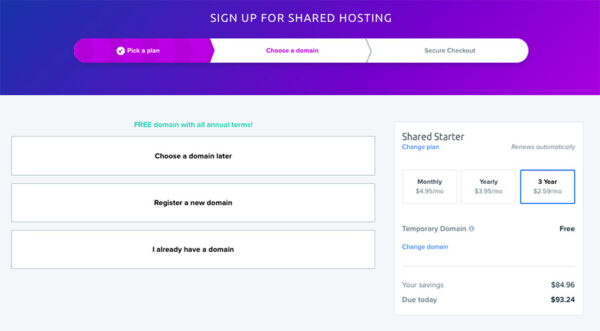The image showcases a webpage header featuring a gradient background transitioning from blue on the left to purple on the right, with a blend of the two colors in the center. Centered on the header is white text that reads, "Sign up for shared hosting."

Below the header are three interconnected tabs. The first tab, labeled "Pick a Plan," is highlighted in pink. The second tab, "Choose a Domain," appears in pink text on a white background. The third tab, "Secure Checkout," is in grey text on a white background.

Near the bottom left of the page, green text announces, "Free domain with all annual plans." Below this announcement are three white buttons with black text. The first button, highlighted in pink, states, "Choose a domain later." The second button says, "Register a new domain." The third button indicates, "I already have a domain."

On the right side, there are several options and details listed:
- "Share Starter"
- "Change Plan"
- "Renew Automatically"

There are pricing options for three durations: monthly, yearly, and three years, all outlined in blue. Additionally, there's a note about a "temporary domain" being free. A blue button labeled "Change Domain" is present below this information.

At the bottom of the section, it states, "Your savings: $84.96," followed by "Due today: $3.24."